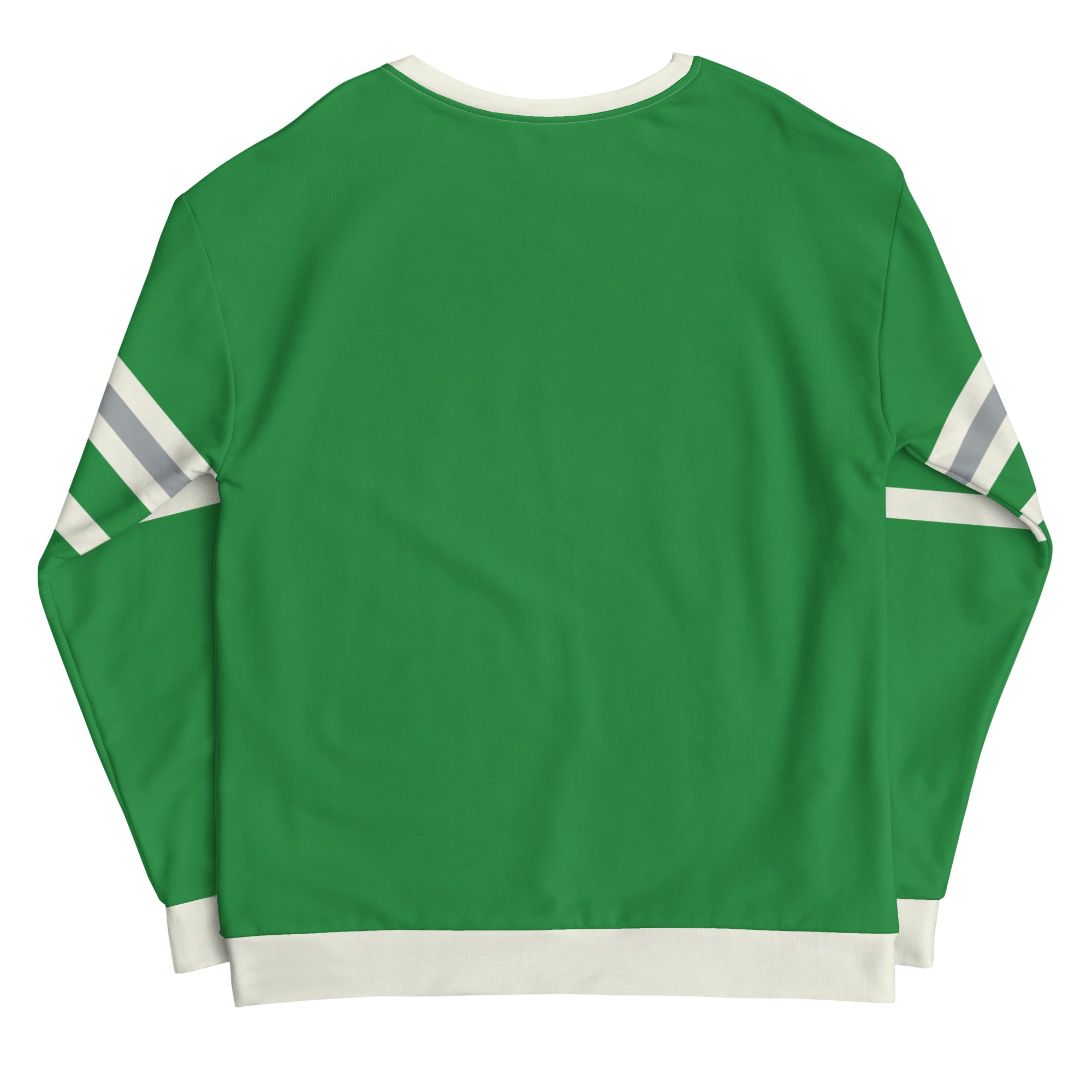The image features a green, long-sleeved football jersey sweatshirt against a completely white background. The sweatshirt has a round crew neck accented by a white band, and similar white bands also accent the cuffs and the hem at the bottom. The sleeves, which are folded with the arms crossed in front and the lower arms placed at the back, showcase a unique pattern: each sleeve is adorned with parallel stripes consisting of a thicker green band flanked by thinner gray and white lines. The main body and the dominant color of the shirt is green, consistent with the stripes on the sleeves. The shirt is notably wrinkled, adding texture to the fabric. There are no visible buttons or other embellishments, and the design appears to lean towards a more masculine aesthetic due to its sporty style.